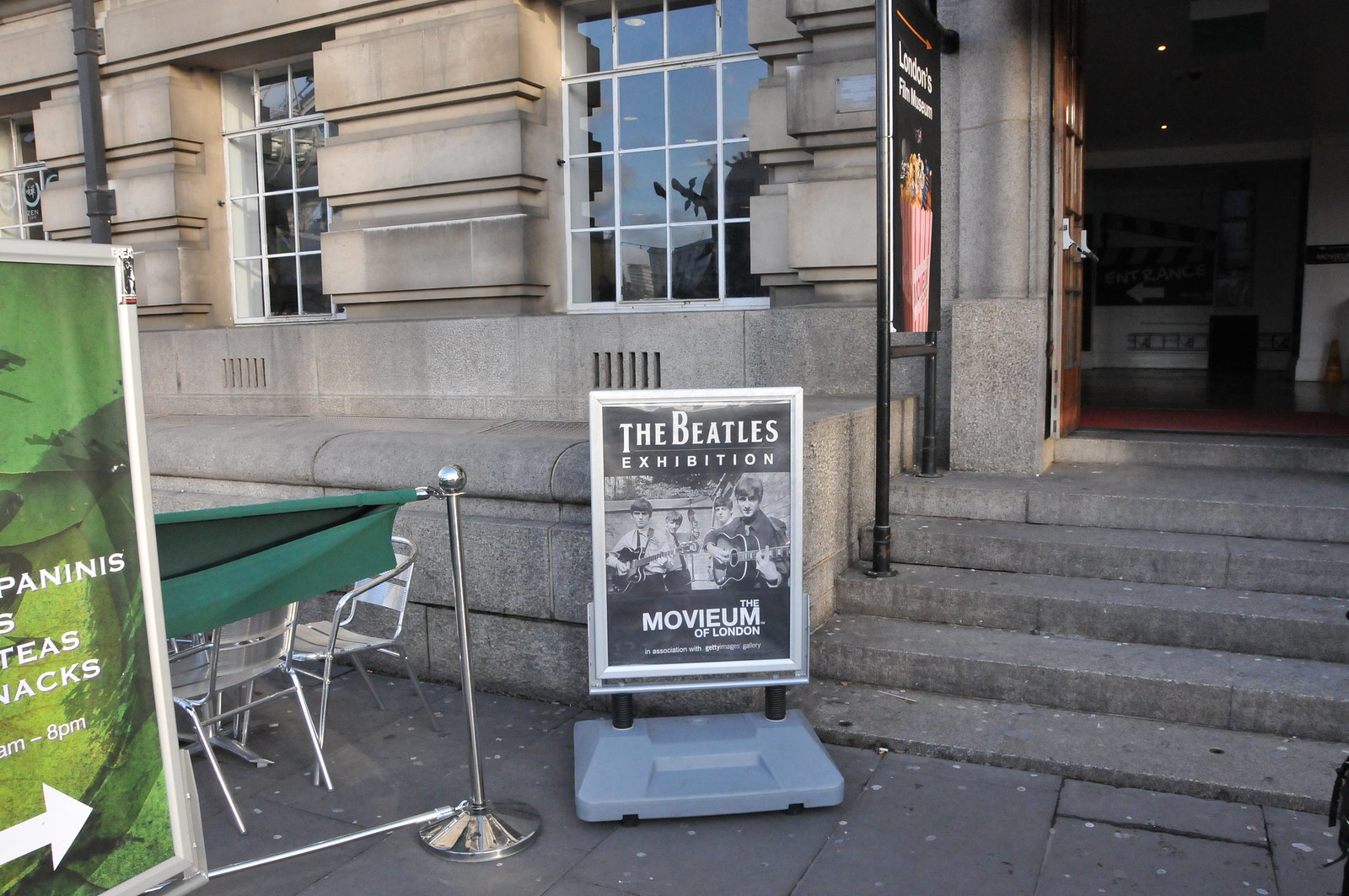This image captures a scene outside a multi-walled stone building featuring open wooden doors and steps leading up to the entrance. Dominating the visual is a black, white, and gray poster advertising "The Beatles Exhibition" with the addition of "Muvium of London," alongside an early career photograph of the iconic band members playing guitars. Positioned prominently near gray, cement-like steps, the poster stands supported by a gray receptacle with two poles. Adjacent to the steps is a fenced seating area with tables and silver chairs. A secondary green-background sign nearby lists "Paninis, Teas, Snacks" and features an arrow pointing towards the main exhibition area. The palette of the image includes various hues like black, white, gray, green, blue, brown, and red, contributing to the detailed and vibrant setting of the photo.